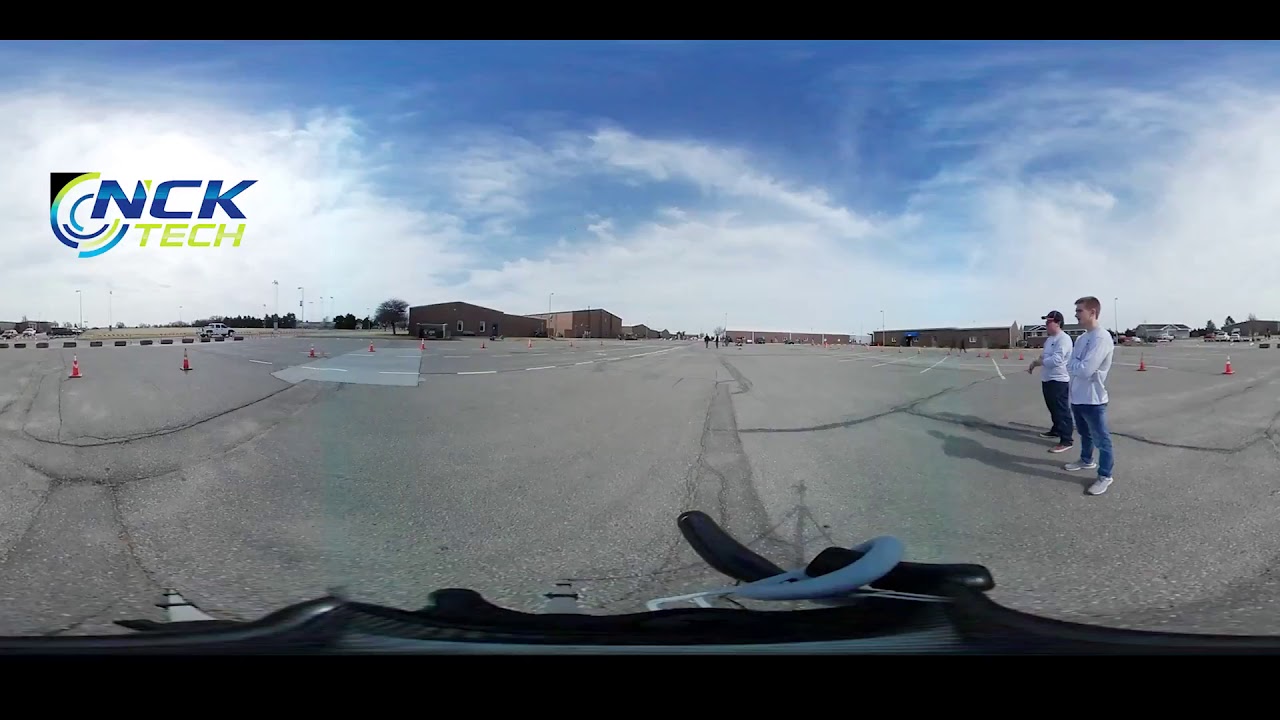The image captures an outdoor setting, likely a test track or parking lot, under a clear, partly cloudy sky in the middle of the day. The ground is made of asphalt, typical of a standard road or racing track. The perspective of the image appears to be distorted by a fisheye lens or 360-degree VR imaging, creating a slight warping effect. In the bottom right corner, there are two men dressed in light shirts and dark pants, standing near several orange and lime green cones scattered across the area. In the upper left corner, there is a computer display featuring the NCK Tech logo in green and blue. The image is framed by a black rectangle, possibly indicating it was captured using a smartphone or tablet on a tripod. In the distance, large buildings can be seen, and there are no visible vehicles except possibly in the far distance on the right. The setting suggests it could be a training or testing area for vehicles, though no vehicles are immediately visible.